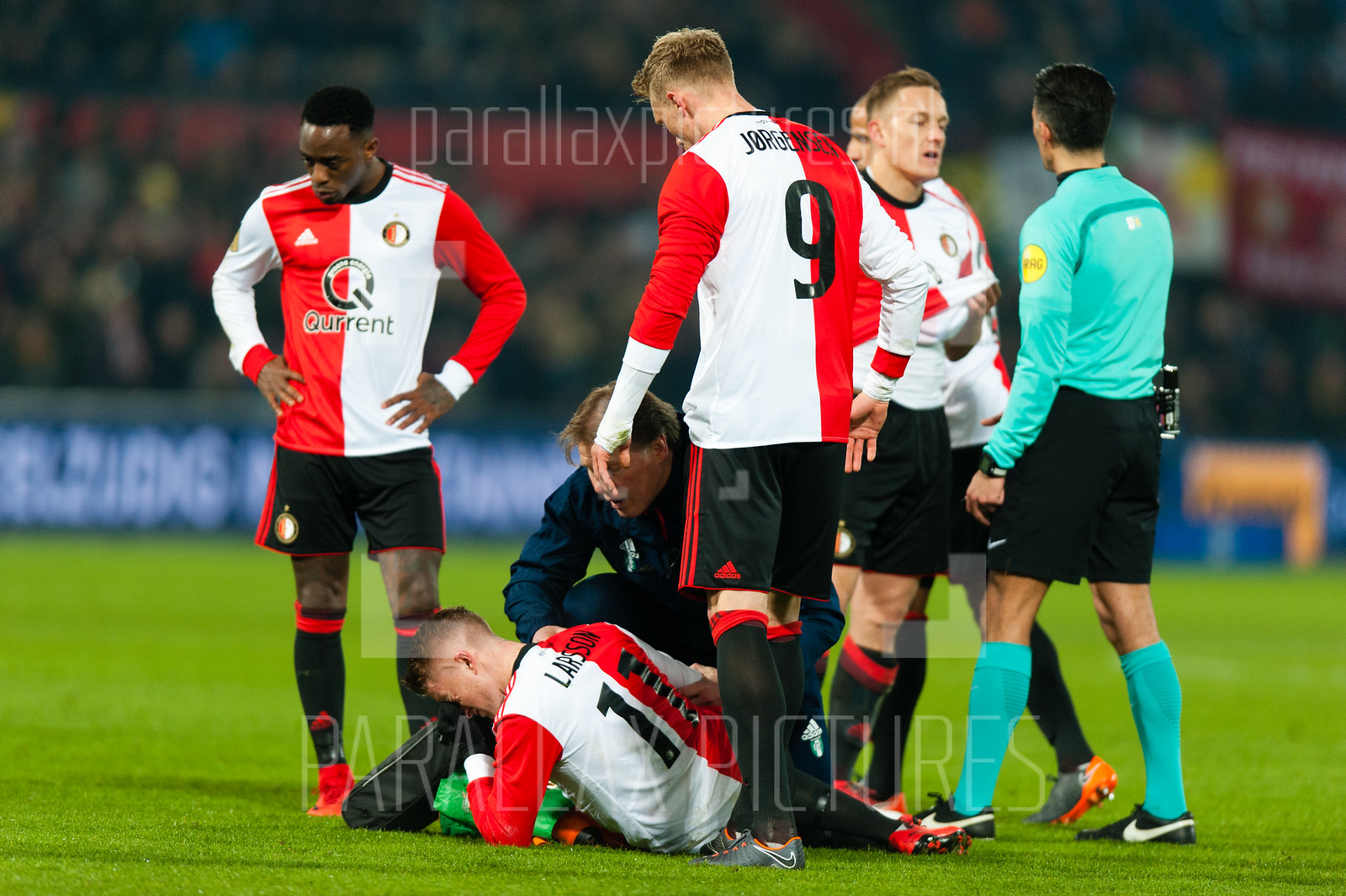The image depicts an intense soccer match on a vibrant green turf field. A dramatic moment has unfolded as one player, wearing a half-red, half-white long-sleeve jersey with the number 11 and the name "Larson" on the back, lies on the ground, seemingly injured. His teammates, identifiably wearing matching red and white jerseys labeled "Q-U-R-R-E-N-T," black Adidas shorts with red piping, and Nike shoes, anxiously surround him. One player, possibly a referee, stands out in a light green long-sleeve jersey, green socks, black pants, and a watch on his left hand, attentively observing the scene. A concerned man in a blue jacket, likely a coach, kneels down, engaged in a focused conversation with the injured Larson, who is visibly in pain. The blurred background reveals the edges of the field, a blue wall with indistinct writings, and an impression of numerous spectators in the stands, adding to the tension and drama of the moment.